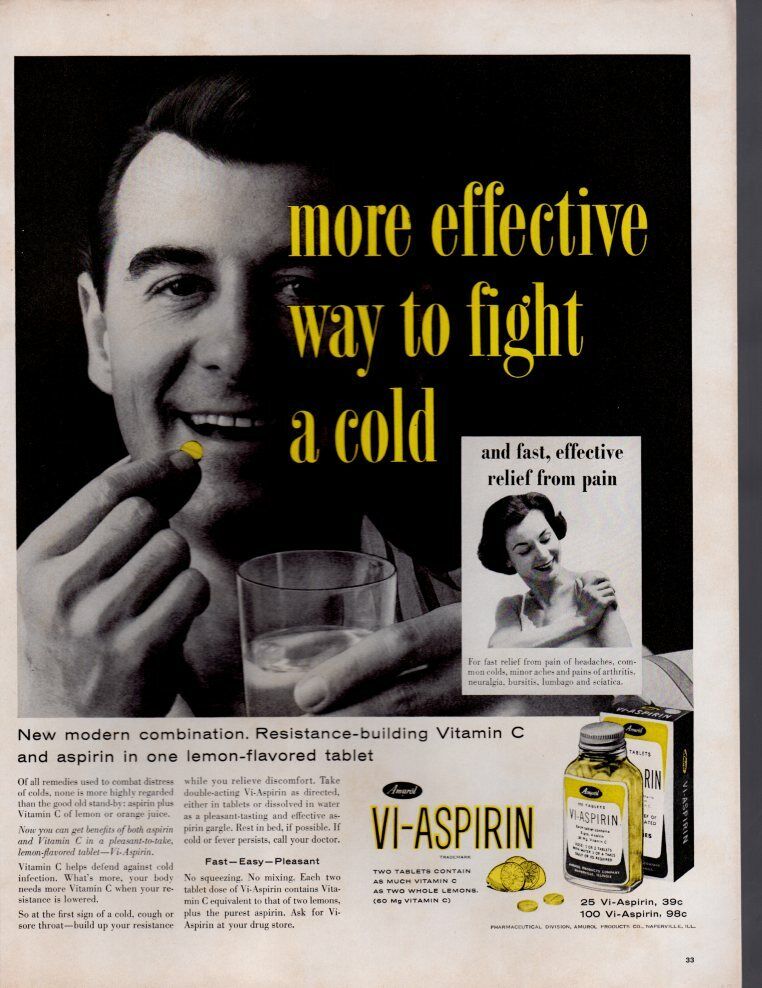This is a detailed advertisement from an older magazine, predominantly in black and white with strategic use of yellow. The main image features a smiling Caucasian gentleman, partially shadowed, with short black hair. He’s in the midst of taking a yellow pill with his right hand and holding a glass of water with his left. Overlaid on the shadowed section of his face are large yellow letters that state, “More effective way to fight a cold.”

Adjacent to this image, there is a white box featuring a woman with a 50s-style short black haircut, dressed in a white camisole or tank top. She appears to be gripping her left shoulder with her right hand. The text over her image reads, “and fast, effective relief from pain,” in black letters.

Below these images, there’s black text describing the product: “New Modern Combination, Resistance Building Vitamin C and Aspirin in One Lemon Flavored Tablet.” Additional paragraphs of text provide more details, though they are not entirely legible. A black-and-white logo in an oval shape displays the product name, Vi-Aspirin, in bold text with a yellow border. Next to this, an illustration depicts some lemons, yellow tablets, and a bottle with a metal screw cap. The bottle, labeled in yellow and black, and the tablets are placed in front of a matching box. This section also includes pricing information right above the page number 33, indicating costs for different quantities of Vi-Aspirin: “25 V.I. aspirin, 39¢. 100 V.I. aspirin, 98¢.” The text also emphasizes that two tablets contain as much vitamin C as two whole lemons.